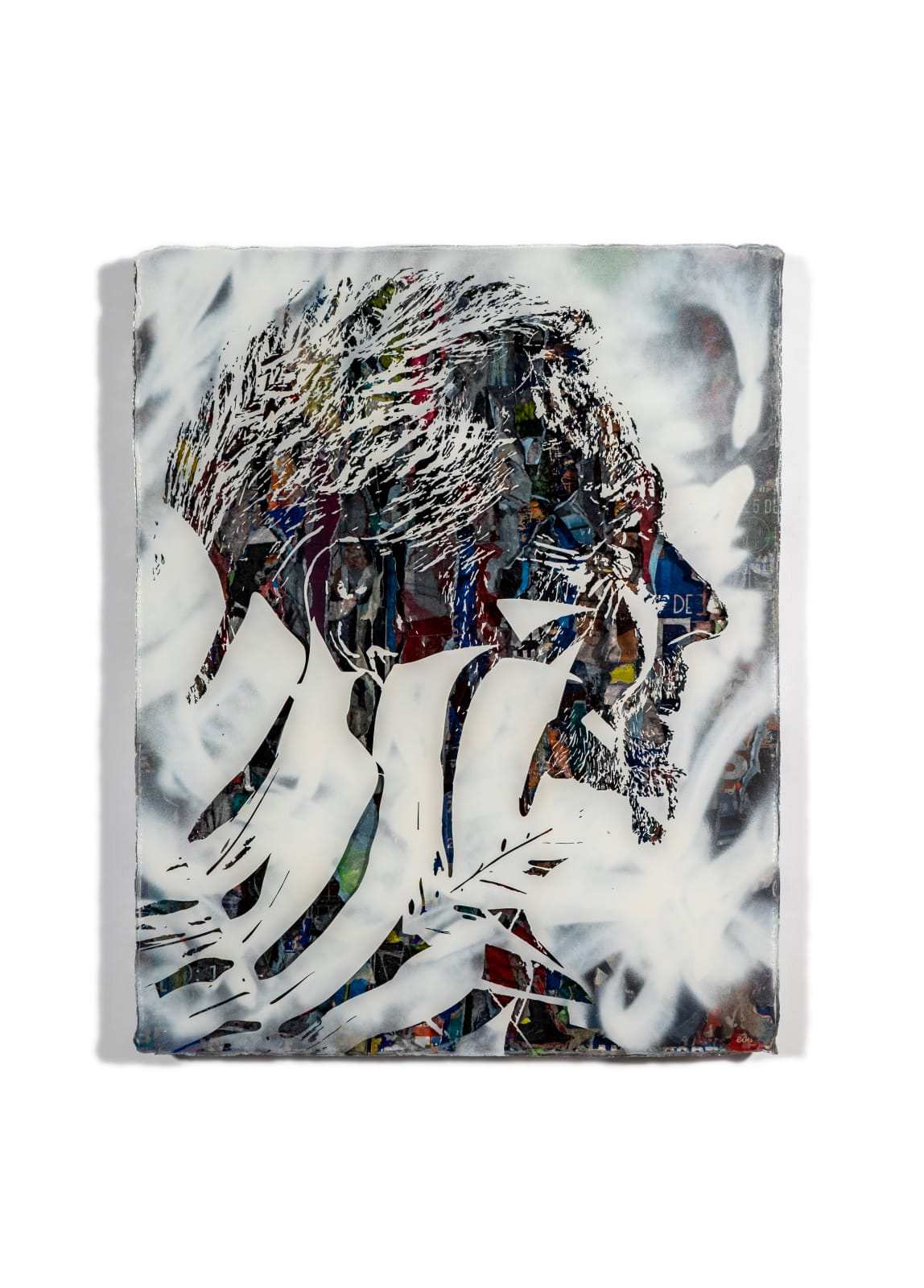This impressionistic artwork presents a detailed profile of a man’s face turned towards the right. The face is created with an abstract amalgamation of colors often associated with impressionist art, blending hues of dark red, gray, dark blue, and black. Unique to this piece is the reversed black and white technique: the shadowed sections of the face, normally black, are rendered in white, while the typically white sections are depicted in black, creating a striking visual effect.

Further enhancing the abstract quality, the man’s hair and facial hair—encompassing frosty white and black lines—add to the textural complexity. The chin and cheek areas exhibit a similar pattern, heavily layered with colors and lines. A notable feature is a white ribbon-like overlay, resembling paint, which covers much of the bottom half of the head.

Embedded within the head’s contours are impressionist representations of various objects and surfaces, possibly hinting at city life. The background continues this theme, supporting a chaotic yet cohesive palette. Lastly, large stripes at the bottom left of the image add an additional layer of intrigue to this multi-faceted portrait.